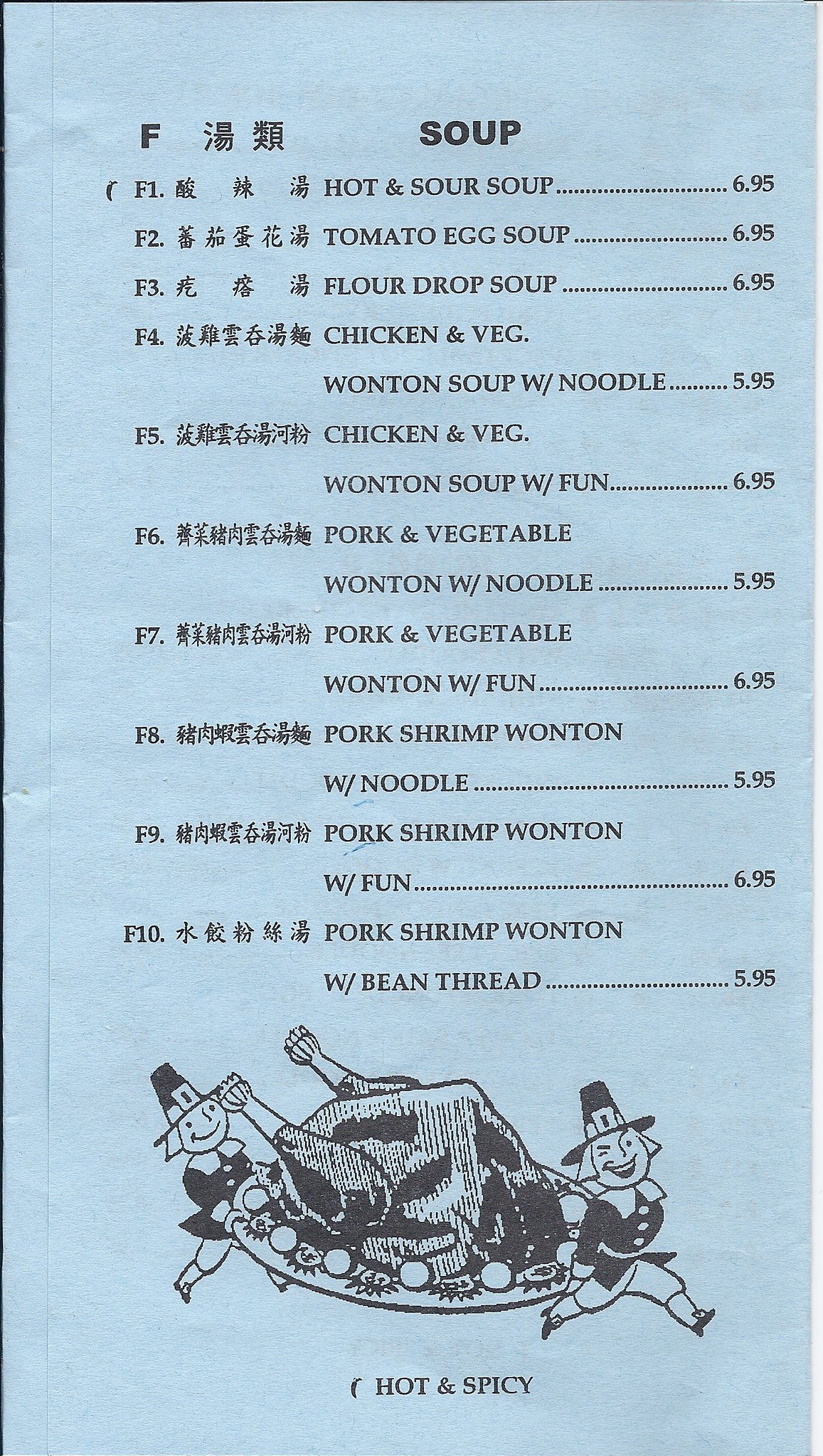This image displays a menu from a Chinese restaurant, specifically from section F, which is dedicated to soups. The page features both English and Chinese text, and it is themed with a light blue background. The section title, "Soup," is prominently displayed in bold at the top, while the soup options are listed below in a standard, smaller typeface.

The menu offers a total of 10 soup varieties, including Hot and Sour Soup, Tomato Egg Soup, and Flour Drop Soup. Among the intriguing options, there is a Pork Shrimp Wonton Soup described with "W/fun" and a Pork and Vegetable Wonton Soup with noodles. Additionally, there's Chicken and Vegetable Wonton Soup with the same "fun" notation, indicating some element of enjoyment or an ingredient called "fun."

Adding a whimsical touch to the menu, the bottom of the page features a cartoon illustration of two smiling pilgrims carrying a large platter with a Thanksgiving turkey, a curious and unexpected detail on a Chinese menu.

Overall, the menu page is a blend of cultural elements and clear, organized listings, catering to both English and Chinese-speaking diners.